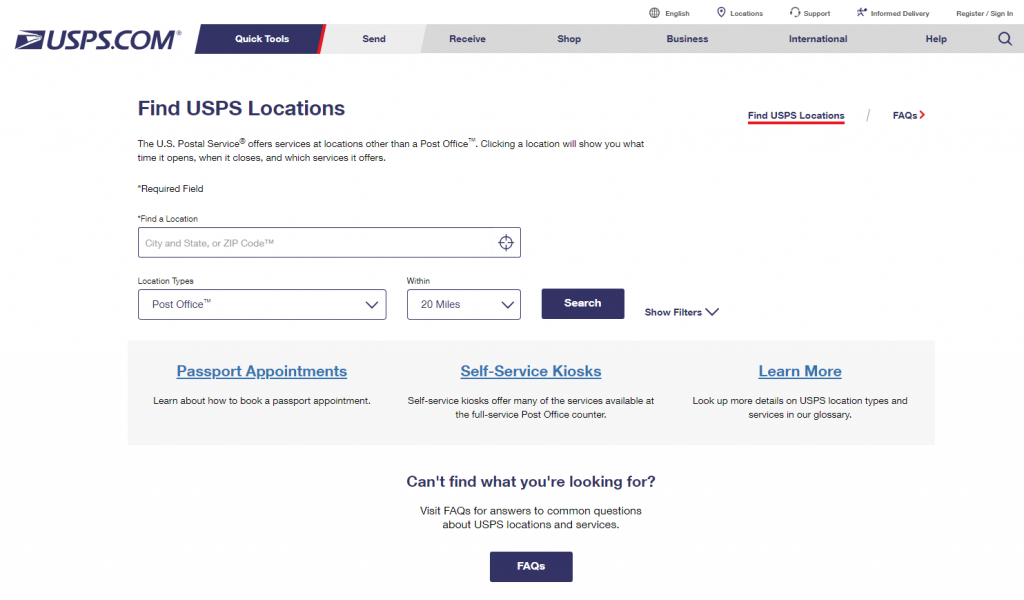The top right corner of the webpage features various menu options in black text, including "English," "Locations," "Headphone Support," "Informed Delivery," and "Register/Sign In." Below these options, on the top left corner, there is a navy blue section that displays "ups.com." This section includes multiple tabs, with the first tab being highlighted in blue with a red line at the end, indicating that it is the currently selected tab. This tab is labeled "Quick Tools" in white text. Other tabs are grey and labeled in navy blue text as "Send," "Receive," "Shop," "Business," "International," and "Help." A navy blue magnifying glass icon is also present.

Below the tabs, there is a navy blue header that reads "Find USPS Locations." The main text body in black explains that "The UPS Postal Service offers services at locations other than the post office. Clicking a location will show you the opening and closing times as well as the services offered." On the right side of this section, underlined in red, it says "Find UPS Locations / FAQs," accompanied by a red arrow pointing to the right.

Further down, the next section prompts "Find Location" and provides a search interface. A rectangular box with a navy blue outline and a white interior asks for "City and State or ZIP Code" in light gray text. Another dropdown menu labeled "Location Type" defaults to "Post Office" and allows the selection of a 20-mile radius. Finally, there's a gray box with navy blue blocks and white text that says "Search."